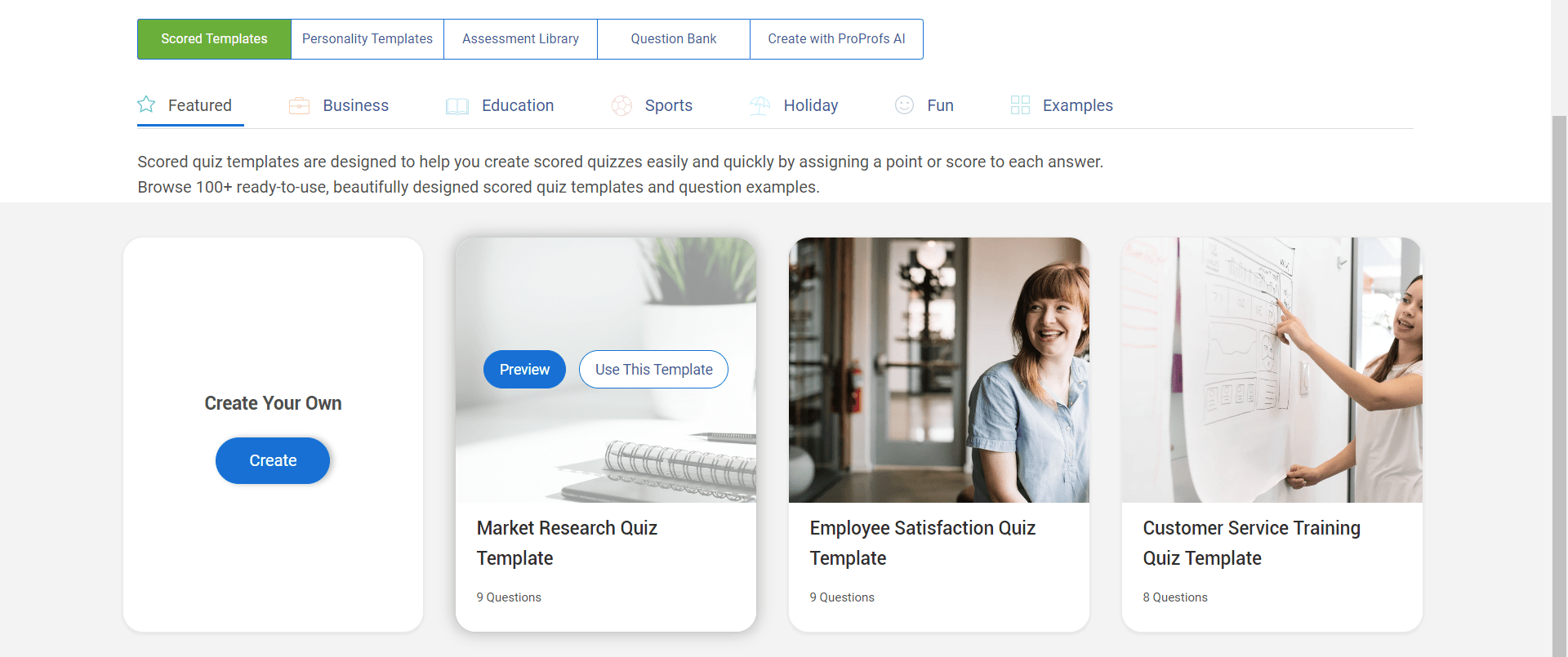This image showcases a webpage tailored for creating assessments and quizzes using ProProfs. Prominently displayed are several linked categories, including "Scored Templates," "Personality Templates," "Assessment Library," "Question Bank," and "Create with ProProfs AI." Additionally, thematic tags like "Future," "Business," "Education," "Sport," and "Holiday" offer varied contexts for quiz creation.

The "Scored Quiz Templates" section is highlighted, emphasizing its purpose to streamline the process of developing scored quizzes by assigning points to each answer. This section boasts over 100 beautifully designed, ready-to-use templates and numerous question examples. Options to "Create Your Own" quiz, preview existing templates, or utilize specific solutions such as "Employee Satisfaction Quiz Templates" and "Customer Service Training Quiz Templates" are also featured. This resource-rich page is designed to facilitate efficient and effective quiz creation for diverse needs.